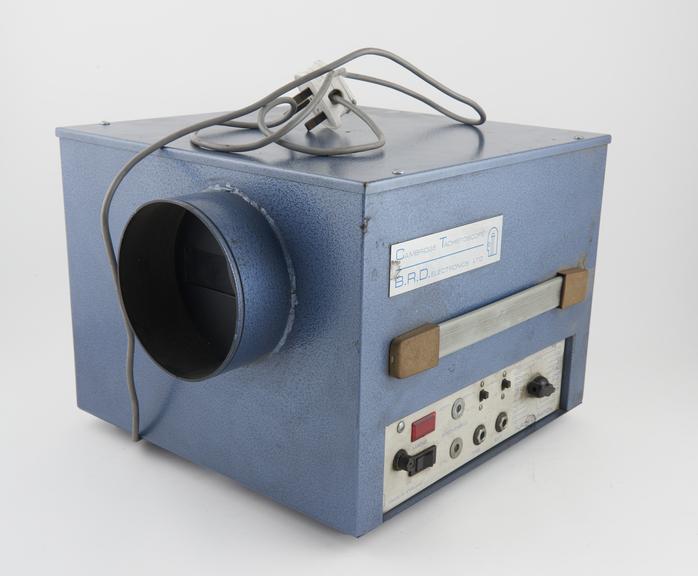The image depicts a blue metal box with various intricate features suggestive of an electronic device, possibly a battery charger or similar equipment. Viewed from an angle, it reveals a gray electrical cord extending from the bottom, equipped with a visible two-pronged plug. The box exhibits multiple connection ports on its sides, intended for plugging in various components. Prominently, a large, round hole with a black interior and a metallic sleeve is visible on one side. The top side features a silver or metallic plaque partially readable, displaying the letters "BRD," alongside another strip that may function as a handle, consisting of a brown-ended, off-white center piece. Additionally, a control panel on the front includes a red button, a black switch for on/off control, multiple plug-in points, a dial, and at least two buttons, further highlighted by a red light indicator. The entire setup suggests utility in connecting and controlling electrical or electronic components, though its exact purpose remains unidentified.